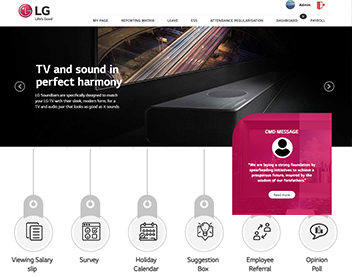This small screenshot of a web page features a dark black bezel at the top, containing barely legible, blurred text. Despite attempts to zoom in, the text remains difficult to decipher. The central portion of the screenshot showcases various images. Notably, there is a large tan building with gray accents in the foreground. Another structure, a lighter tan building with brown elements, includes a prominent fountain area encircled by a gray ring. Adjacent to this, a cluster of homes with dark and light green lawns is visible.

Beneath these images, each is accompanied by two buttons: a white one with black text, and a dark gray one with white text. Several sets of images are displayed, including one featuring a brown and tan building, another with a yellow and white building, and yet another with a brown and red building.

On the left-hand side, there are the names of three locations: "ITC Grand Chola" (with the exact words partially obscured), "Martha Mumbai," and "Grand Central Mumbai." At the top left, within a hard-to-read dark gray bezel, there are three lines symbolizing settings. Additionally, on the top right within a secondary light gray section, there is a dark gray button.